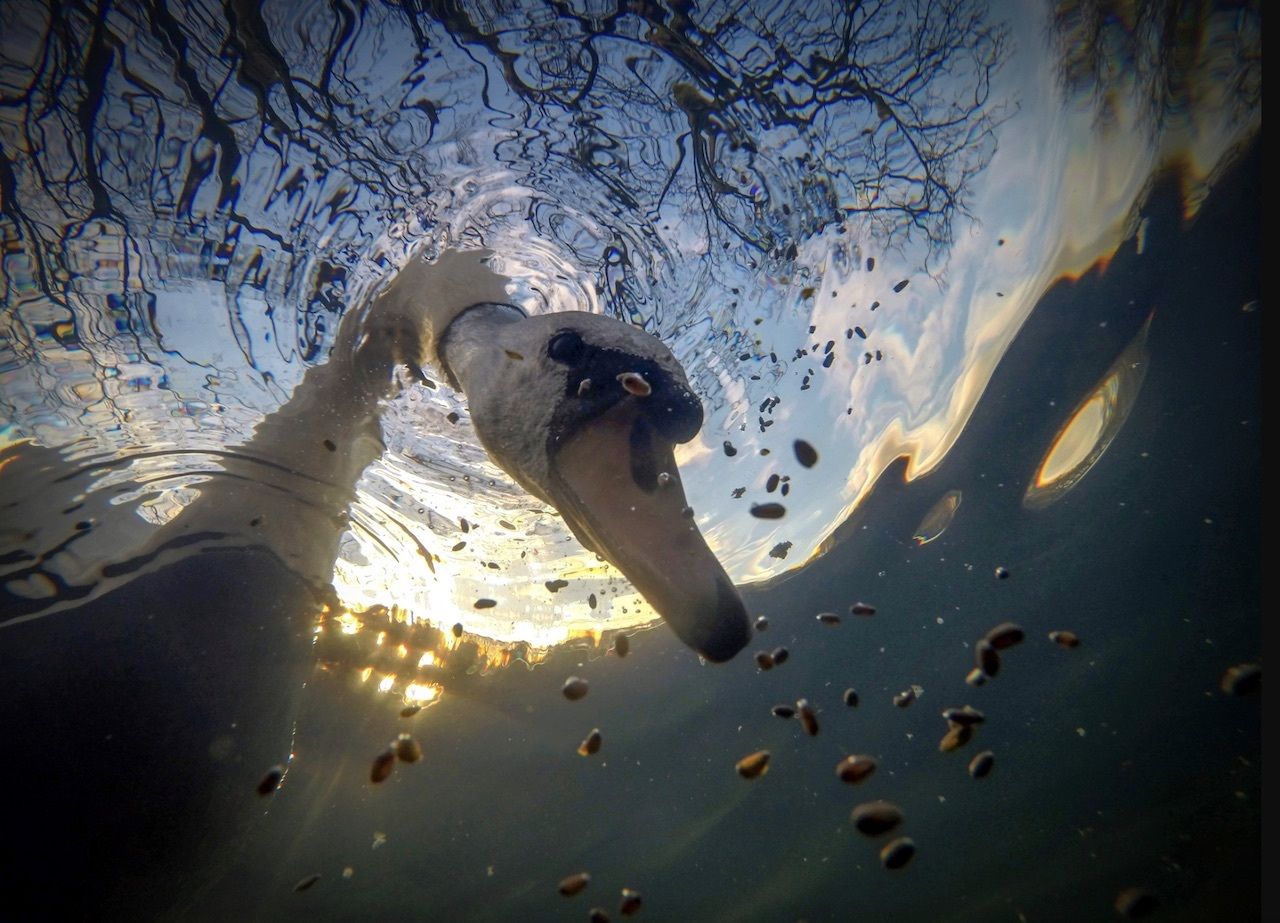In this captivating underwater image, a duck with a distinctive white head and black markings around its beady eyes is seen dipping its head through the surface of a blue, sunlit body of water. The duck is actively foraging for small, round pellet-like seeds that are scattered and floating around. The sunlight highlights ripples emanating from the duck's submerged head, adding a dynamic texture to the scene. Above, the silhouettes of tree branches are discernible against a backdrop of a clear blue sky with scattered white clouds, while beams of sunlight filter through, illuminating the duck’s activity. The nuanced details, such as the duck’s open beak and the gritty sponge-like marks at the bottom right, add depth to this stunning and peaceful aquatic moment.